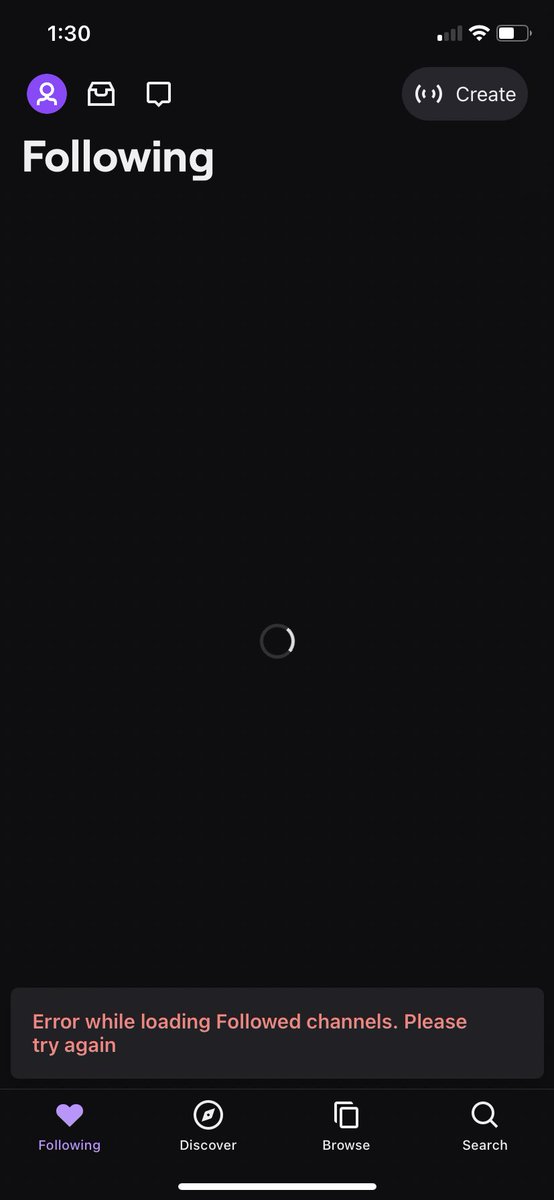The image is a screenshot from a cell phone interface, displayed in a vertical rectangular format with a black background. At the top left corner, the time is shown as 1:30. Adjacent to the time in the top right are icons for Wi-Fi connectivity and battery status. Directly below the time on the left, there's a purple circular icon with a white line drawing resembling a person. To the right of this icon, there is an image of a white box followed by a square speech bubble icon. Beneath the battery symbol on the far right, there is an oval button labeled "Create."

Underneath these top icons, the word "Following" is displayed on the left side. The main body of the image is empty except for a small circular icon located in the center. This circle is predominantly gray with a small white segment, suggesting a spinning or loading animation.

At the bottom of the image, a gray bar contains a message in pink text: "Error while loading. Followed channels. Please try again." Finally, at the very bottom left corner, a purple heart icon is displayed with the word "Following" next to it.